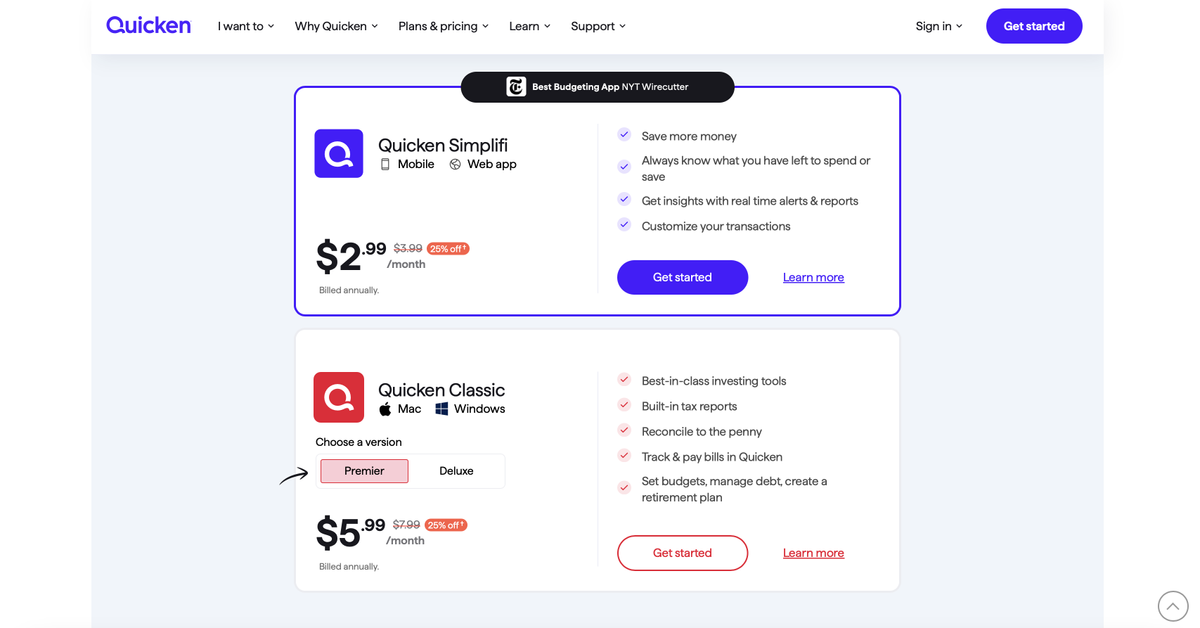The image is a screenshot of the Quicken website's purchase page for their software. At the top left corner of the page, the word "Quicken" is displayed in bold blue text. Directly below it, there's a white rectangular box bordered in blue, featuring the text "Quicken Simplify Mobile web app $2.99 per month." Adjacent to the price, a small red banner with white text indicates a 25% discount. On the right side of this section, several key benefits are listed: 

- Save more money
- Always know what you have left to spend or save
- Get insights with real-time alerts and reports
- Customize your transactions

Beneath these points, there is a blue oval banner with white text stating "Get Started."

Below this section, there's an option for "Quicken Classic," which allows the user to choose between Mac or Windows versions. The user must then select a version, with two options presented in a pink rectangular box with black text: "Premier" or "Deluxe." The pricing for these options is shown with the original price of $5.99 and $7.99 crossed out in red, indicating a current discount. Another red banner nearby reiterates the 25% discount. To the right of this information, the advantages of selecting this product are provided. At the bottom of this segment, there is a white button with red text that says "Get Started."